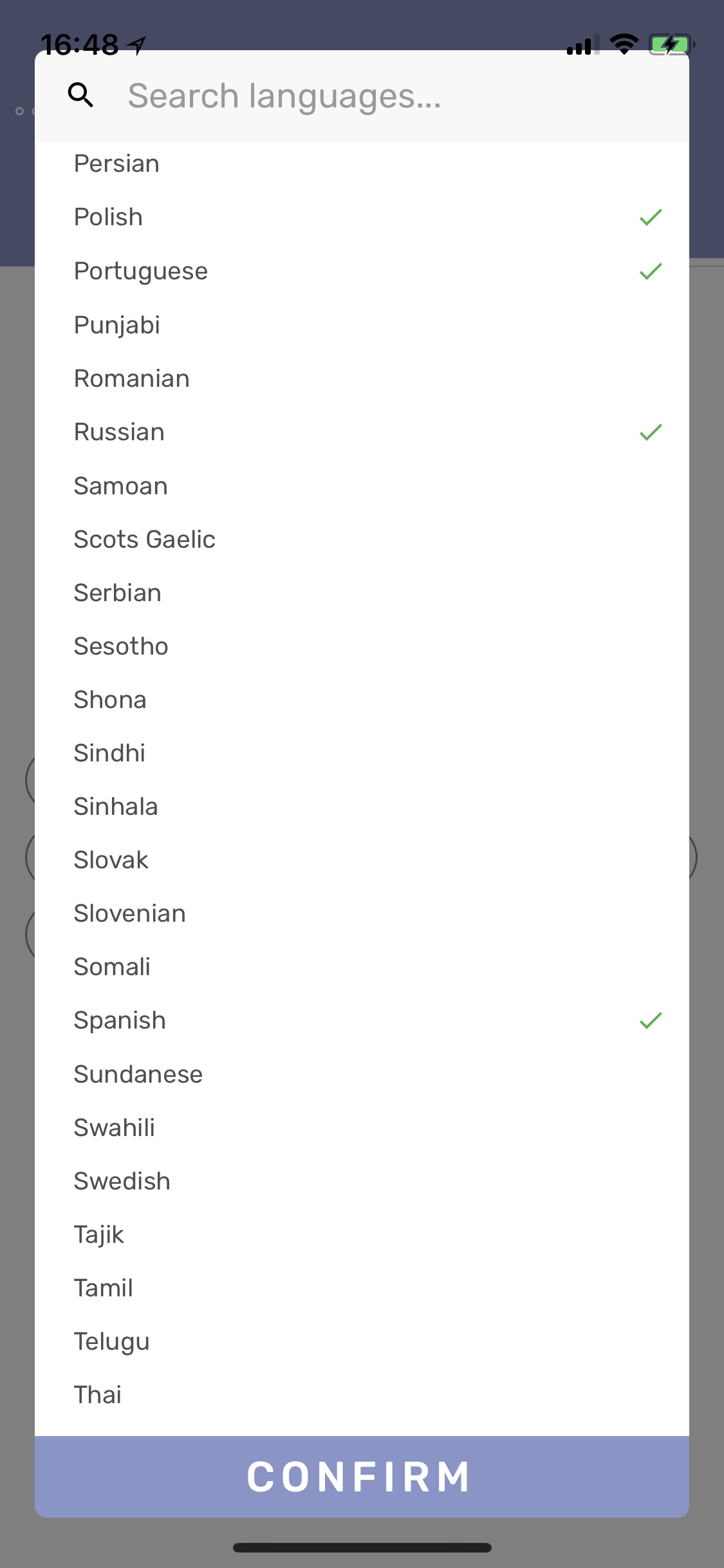This screenshot captures a cell phone screen displaying the available language settings menu. The phone is actively charging, as indicated by the battery icon showing a charging symbol, and it is also connected to Wi-Fi with a signal strength of 3 out of 4 bars. The screen specifically focuses on a search bar used for searching language options. Displayed right below it are multiple languages available for selection, including Persian, Polish, Portuguese, Punjabi, Romanian, Russian, Samoan, Scots Gaelic, Serbian, Sesotho, Shona, Sindhi, Sinhala, Slovak, Slovenian, Somali, Spanish, Sudanese, Swahili, Swedish, Tajik, Tamil, Telugu, and Thai. The crisp, clear image provides a detailed view of the phone's interface and its current operational status.